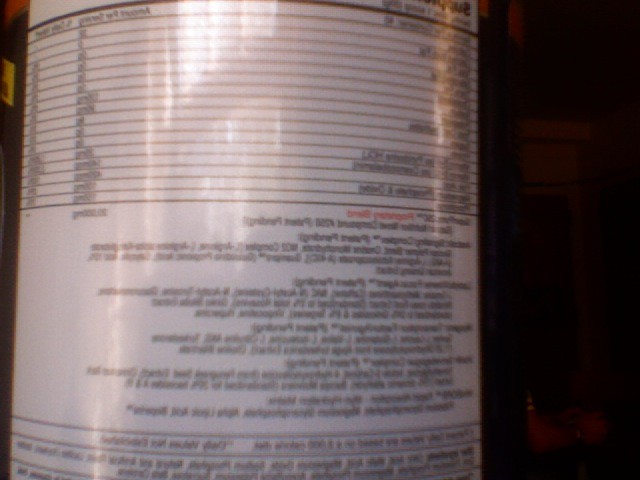This photograph captures a large bottle, seemingly filled with pills, potentially vitamins, standing prominently in the foreground. The bottle is covered with several lines of text detailing its contents, though the small print renders it illegible. To complicate matters, the image appears to be mirrored, making the text even harder to decipher. The setting appears to be within a dimly lit house, possibly illuminated by sunset light or a warm, orange-hued lamp. In the background, a pair of human hands are visible, gripping what looks like a controller, adding a hint of daily life and modern activity to the composition.